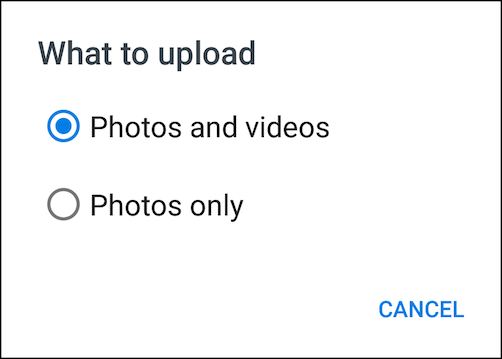The interface appears to be a user prompt for selecting media types to upload. The overall layout is predominantly white, while the edges are outlined in black, giving it a framed, square appearance. In the top left corner, there's a heading in capitalized letters that reads "WHAT TO UPLOAD." Below this heading, there are two selectable options:

1. A circular checkbox that is checked, labeled "photos and videos."
2. A circular checkbox that is unchecked, labeled "photos only."

In the bottom right corner of the interface, there is a blue button labeled "CANCEL." The primary backdrop remains white, offering a stark contrast against the black borders. The interface is designed to guide users in choosing their desired media formats for upload, with clear, distinct options and a minimalistic, straightforward layout.